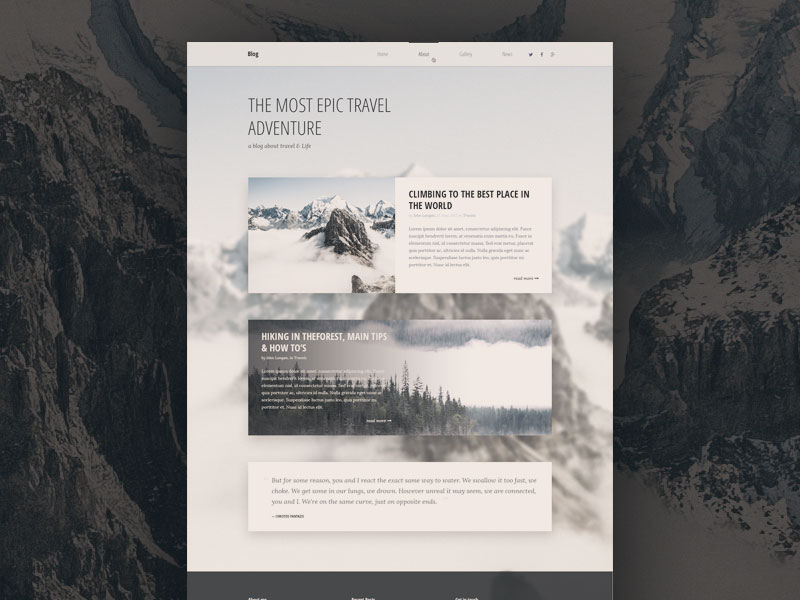Screenshot of a travel website featuring a backdrop of majestic, snow-capped mountains set against a slightly grayish background. An overlay image appears above the background, potentially leading to a blog. At the top left corner, "Blog" is boldly labeled, flanked by other barely legible menu options and several icons to the right.

On the left side, the text "The Most Epic Travel Adventure" stands out, accompanied by a smaller subtitle beneath it. Below this, a media image is captioned "Climbing to the Best Place in the World," followed by a descriptive paragraph. This image showcases towering mountains emerging through a blanket of clouds.

Further down, another segment titled "Hiking in the Forest: Main Tips and How-To's" introduces a comprehensive guide, paired with a scenic photo of a lush forest and expansive sky. At the very bottom, a rectangular box contains an additional paragraph, providing more detailed information.